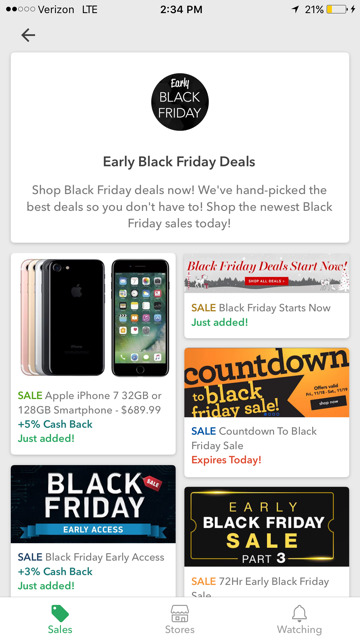### Detailed Caption

The image displays a mobile phone screen with a white background. It is 2:34 p.m., and the battery level is at 21 percent, indicated by a charging thunderbolt symbol. The phone carrier is Verizon, showing LTE connectivity. A back arrow and a black circle icon are also visible.

Prominent text announces "Early Black Friday Deals" in bold letters. Below, it encourages users to "Shop Black Friday deals now" with a message that highlights how carefully selected deals are presented to save the viewer from extensive searching. The featured section includes the latest Black Friday sales, urging immediate action.

A few iPhones are showcased, specifically their backs, except for one flipped over displaying its screen. A prominent tag on the screen reads "SALE" in green. The sale highlights an Apple iPhone 7 with either 32 GB or 128 GB storage, priced at $689.99, plus an additional offer of 5% cash back.

Further text stresses the urgency of the deals with phrases like "Black Friday deals start now," "Just added," and "Countdown to Black Friday sale," with an expiration warning in red. The image also mentions "Black Friday early access" repeatedly, along with a 3% cash back offer for early shoppers.